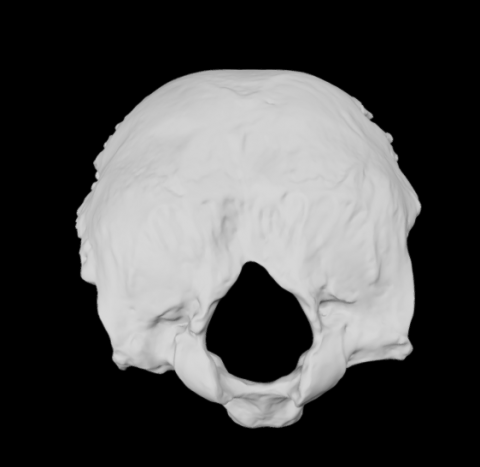The image features a mostly circular, white plaster mold set against a dark, black background. The rough texture of the mold, reminiscent of wrinkles, gives it an organic appearance. A prominent, large, triangular-shaped hole near the bottom center of the mold evokes the resemblance of a skull, particularly the back where the brain would have its spinal cord emerging. This hole looks somewhat like the aperture from a skull, though it may also suggest the likeness of a mushroom cap opening or Hershey Kiss shape. The simplicity of the photograph, with no additional lighting or text, emphasizes the stark contrast between the white plaster and the black surroundings.